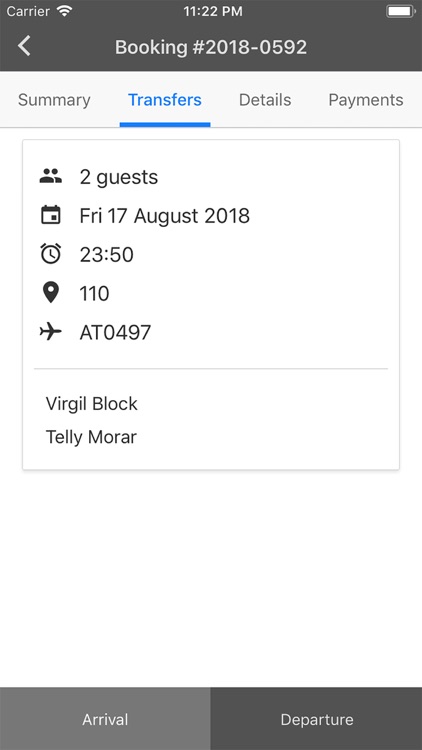The smartphone screen displays a user's booking details with a well-organized layout. At the top, a dark gray banner runs horizontally, showing "11:22 PM" in the center in white text, with a battery icon indicating a full charge to the right, and the word "Carrier" to the left. Directly below, a white text line reads "Booking Number: 2018-0592," accompanied by a back arrow on the left.

Under this, a light gray banner presents a navigation bar with the sections "Summary," "Transfers," "Details," and "Payments." The "Transfers" section is highlighted in bright blue, with a corresponding bright blue line underneath, while the other sections remain in gray text.

Following this banner is a vertical list in black text with accompanying icons: 
- "Two Guests" with a people icon
- "Friday, the 17th, August 2018" with a calendar icon
- "23:50" for time with a clock icon
- "110" with a location icon
- "AT0497" with an airplane icon

A faint gray line separates these details from the names "Virgil Block" and "Telly Morar" in gray text below. At the bottom of the screen, two boxes highlight different sections: "Arrival" in white text inside a light gray box on the left, and "Departure" in white text inside a dark gray box on the right. The overall design is clean and user-friendly, providing clear, concise information for the user.